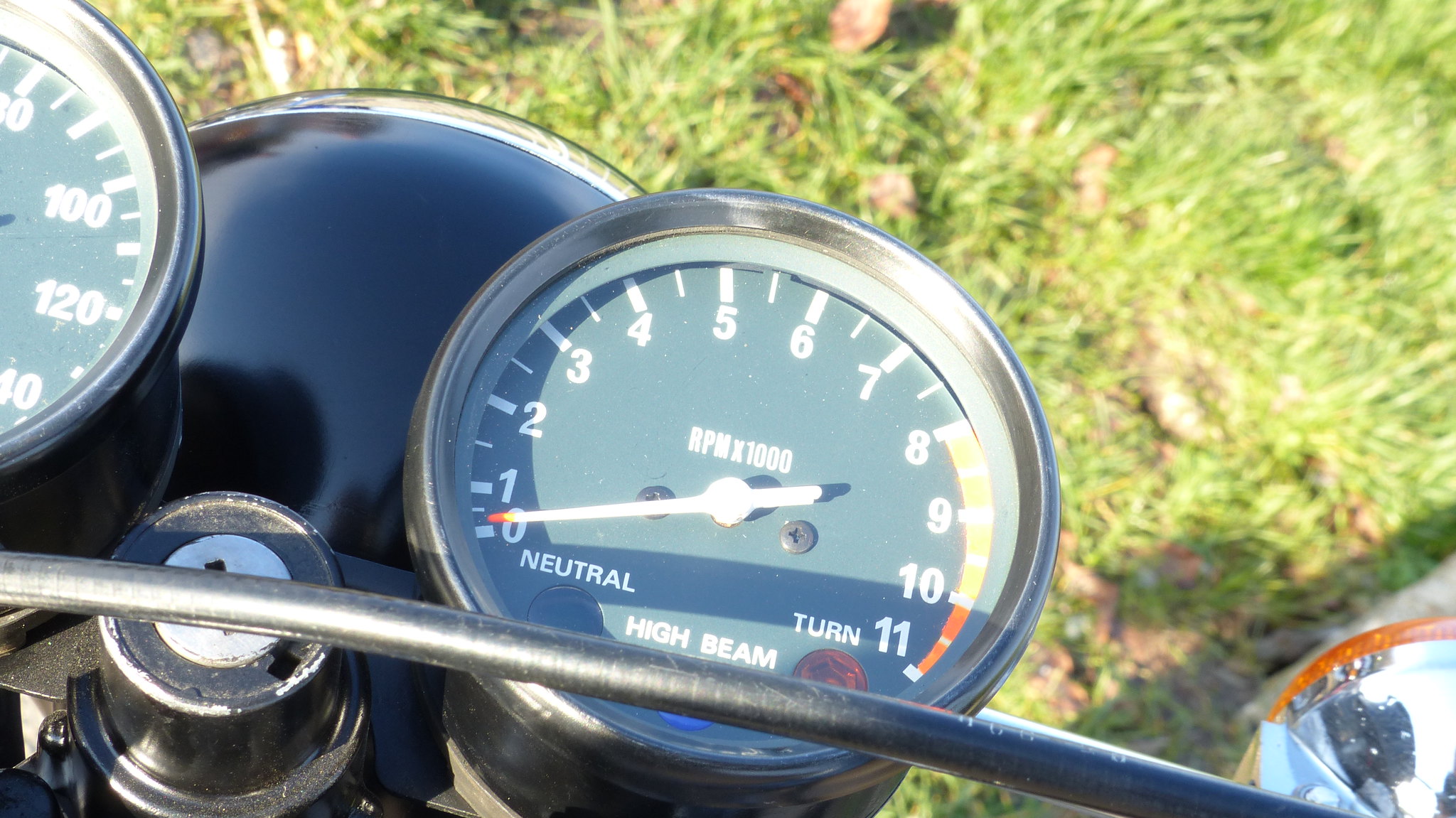This detailed photograph showcases the front of an unknown vehicle, possibly a motorcycle or lawnmower. Central to the image is a circular speedometer-like gauge, displaying numbers ranging from 0 to 11. Below the 0 is the word "Neutral," and below the 11 is the word "Turn." The gauge is color-coded with a yellow segment from numbers 8 to 10, which transitions to orange from 10 to 11. The needle of the gauge is currently resting at 0. Above the midpoint of the dial is the label "RPM x 1000." At the bottom center of this circular gauge, the words "High Beam" are visible. A metallic component traverses below the gauge, and a headlight is positioned in the bottom right corner of the image. The background features slightly out-of-focus grass with scattered old leaves, suggesting a natural, somewhat untidy setting. In the top left of the photograph, a partial view of another gauge is visible, displaying numbers 80, 100, 120, and 140, but further details of this gauge are obscured.